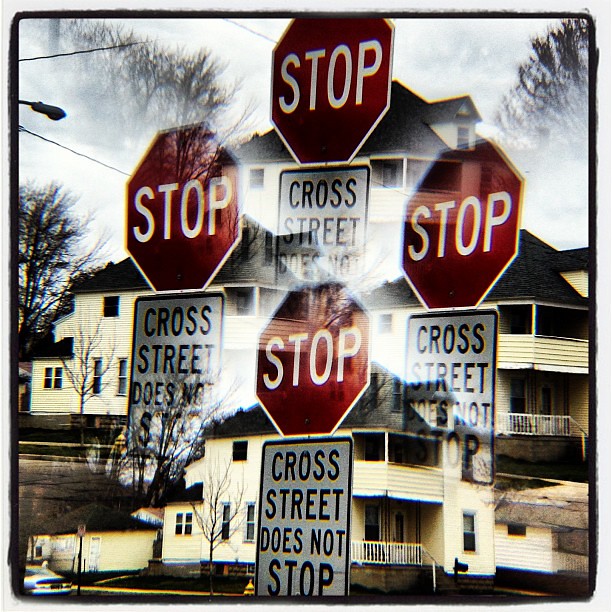In this intricately layered image, a focal white house with a distinctive black roof and a large porch on the top floor draws immediate attention. The house is repeated four times in a diamond shape, overlapping artistically, giving the image a vintage feel as if it were framed by an old photograph. In each instance of the house, a tall tree is visible on the left side, adding a touch of uniformity across the repetitions. The house, which actually has yellowish paneling, features a fenced-in entryway beneath the porch, indicating a two-story structure. 

A bright red stop sign stands prominently in front of the house with a white rectangular sign below reading, "Cross Street Does Not Stop." The image manages to capture a bit of the street, revealing the back of a silver car parked nearby and a yellow house adjacent to the primary white house. Additionally, a small yellow shed peeks out from behind the house, contributing to the layered, almost collage-like composition. A black mailbox is seen at the front, along with a small front porch. To the upper left of the image, a street light stands, illuminating the scene. The overall effect of the repeated, fading images and the subtle foggy cloudiness between them lends a nostalgic, timeless atmosphere to the photo.